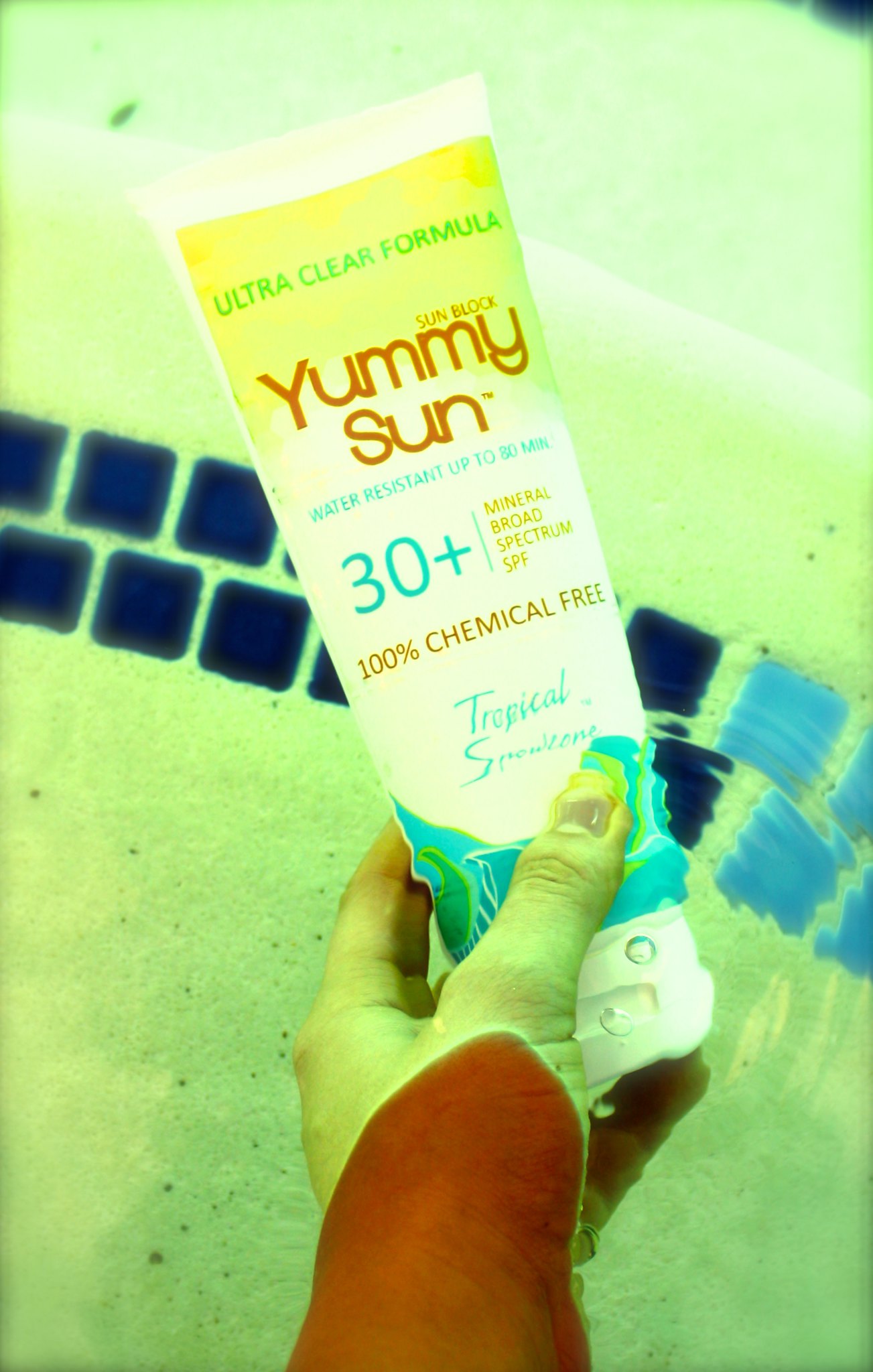The photograph features a tube of sunblock labeled "Yummy Sun," prominently displayed against the backdrop of a pool with a cement bottom adorned with small blue tiles. The tube, primarily white, sports a vibrant label that transitions from yellow at the top, to white in the center, and blue at the bottom. In green text on the yellow section, it reads "Ultra Clear Formula, Yummy Sun, Sunblock." The white center part features blue text that states, "Water Resistant up to 80 Minutes, 30 Plus." Additionally, in yellow text, it reveals "Mineral Broad Spectrum SPF, 100% Chemical Free." The blue bottom section of the label, partly obscured, presumably includes the word "Tropical." The sunblock is held by a hand partly submerged in a thin, shallow layer of clear water, causing the hand to appear greenish due to the water's refraction.